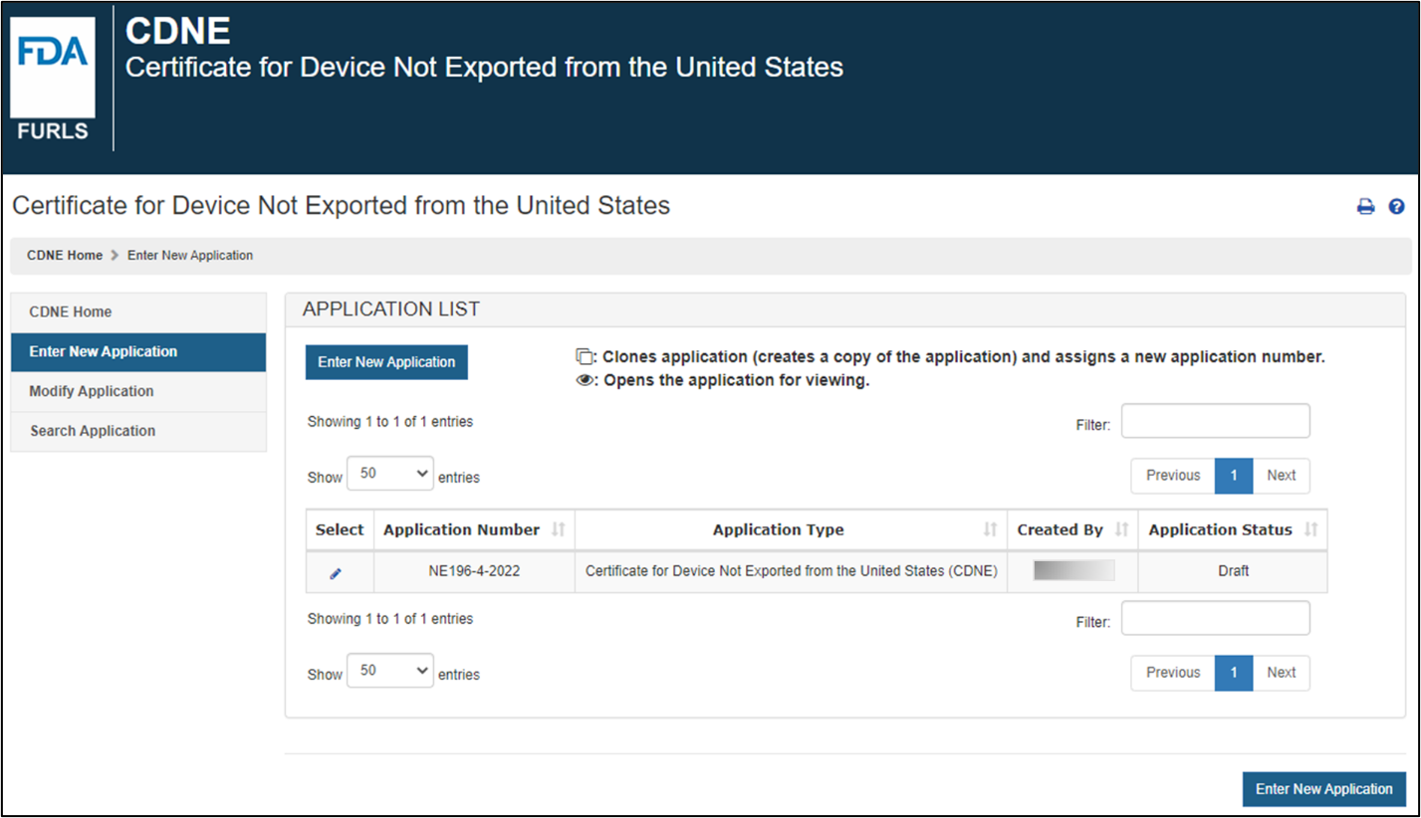On a vivid blue background, the upper left-hand corner features a white rectangle with blue text that reads "FDA," and beneath that, in white text, it says "FURLS." Adjacent to this section, it says "CNDE," followed by the phrase "Certificate for Device Not Exported from the United States" in white text.

On a white background with black text, the words "Certified" or "Certificate for Device Not Exported from the United States" are visible once more. A gray section displays "Black Tex" and "CNDE Home, Enter New Application."

Descending along the left side, there are several categories listed:
- In white on a blue background: "CNDE Home, Enter New Application."
- On black with gray text: "Modify Application," "Search Application," and "Application List."
- In white on a blue background, inside a box: "Enter New Applicant."

Returning to white text on a black background, it reads:
- "Clone Application," describing the process as creating a copy of the application, assigning a new application number, and opening the application for viewing.

Further details describe the selection process for an application, including the application number, type of application, creator (information scratched out), and application status marked as "Draft."

At the bottom right, another blue rectangle with white text says "Enter New Application."

This comprehensive image layout portrays various sections and functionalities related to CNDE data entry and application management on a visually engaging interface.